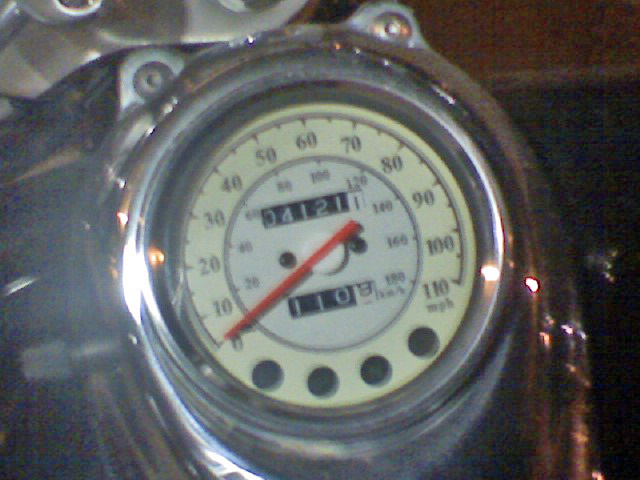The image is a rectangular landscape photograph of a speedometer, which appears to be from a motorcycle, given its design elements. The overall composition is slightly dark and somewhat blurry. Central to the image is a circular speedometer enclosed in a thick silver metallic frame, accentuated by concentric stacking rims. On the top, left, and right edges of this frame are small, flat projections resembling "bunny ears," each secured by visible rivets.

The background is indistinct, providing no clear identifying features. The speedometer face is tilted slightly to the left, about 5 to 10 degrees off the vertical axis, causing its numerical markings to appear angled. The outer ring of the gauge's face is a light yellow, contrasting with the inner white portion. Around this outer ring are numerals incrementing by tens from zero to 110, with "MPH" labeled beneath the 110 mark in lowercase letters. The numbers arc around the dial, covering approximately 280 degrees of the circle, leaving the bottom part devoid of numerical markings.

At the base of the dial, spanning from left to right between the zero and the 110 markings, are four small, black circular shapes, casting shadows that make them appear raised from the surface. A prominent red needle, extending from the center and pointing to zero, is the main indicator of speed.

Above the red needle is an odometer display, featuring black numbers on a white background showing "34121," while below the needle is another measurement reading "110" with a black nine on a white background as the last digit. There is some illegible text adjacent to these numbers. 

Within the white central circle of the gauge, beneath the bold black MPH numerals on the yellow perimeter, are the kilometers per hour readings, also in black numerals on a white background.